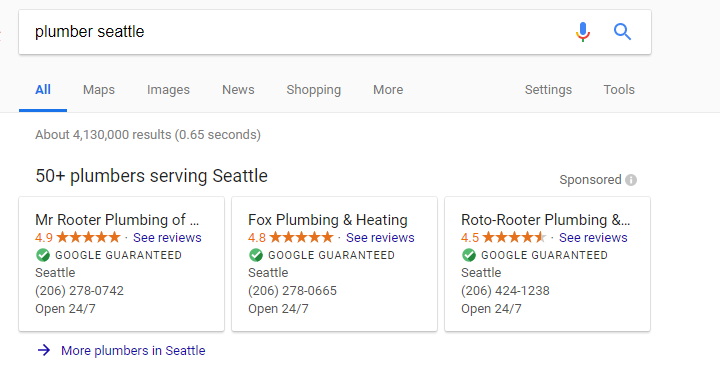The image depicts a Google search results page for "Plumber Seattle." The search bar at the top confirms the query, with the "All" tab selected to display comprehensive results. Google retrieves about 4 million results, indicating the vast number of related pages. The search highlights that over 50 plumbers are available in the Seattle area.

The top three results are prominently displayed within distinct boxes, and all are marked as sponsored ads. These listings include:

1. **Mr. Rooter Plumbing** - Rated 4.9 stars.
2. **Fox Plumbing and Heating** - Rated 4.8 stars.
3. **Roto-Rooter Plumbing & Water Cleanup** - Rated 4.5 stars.

All three businesses operate 24/7, ensuring round-the-clock service for Seattle residents in need of plumbing assistance.